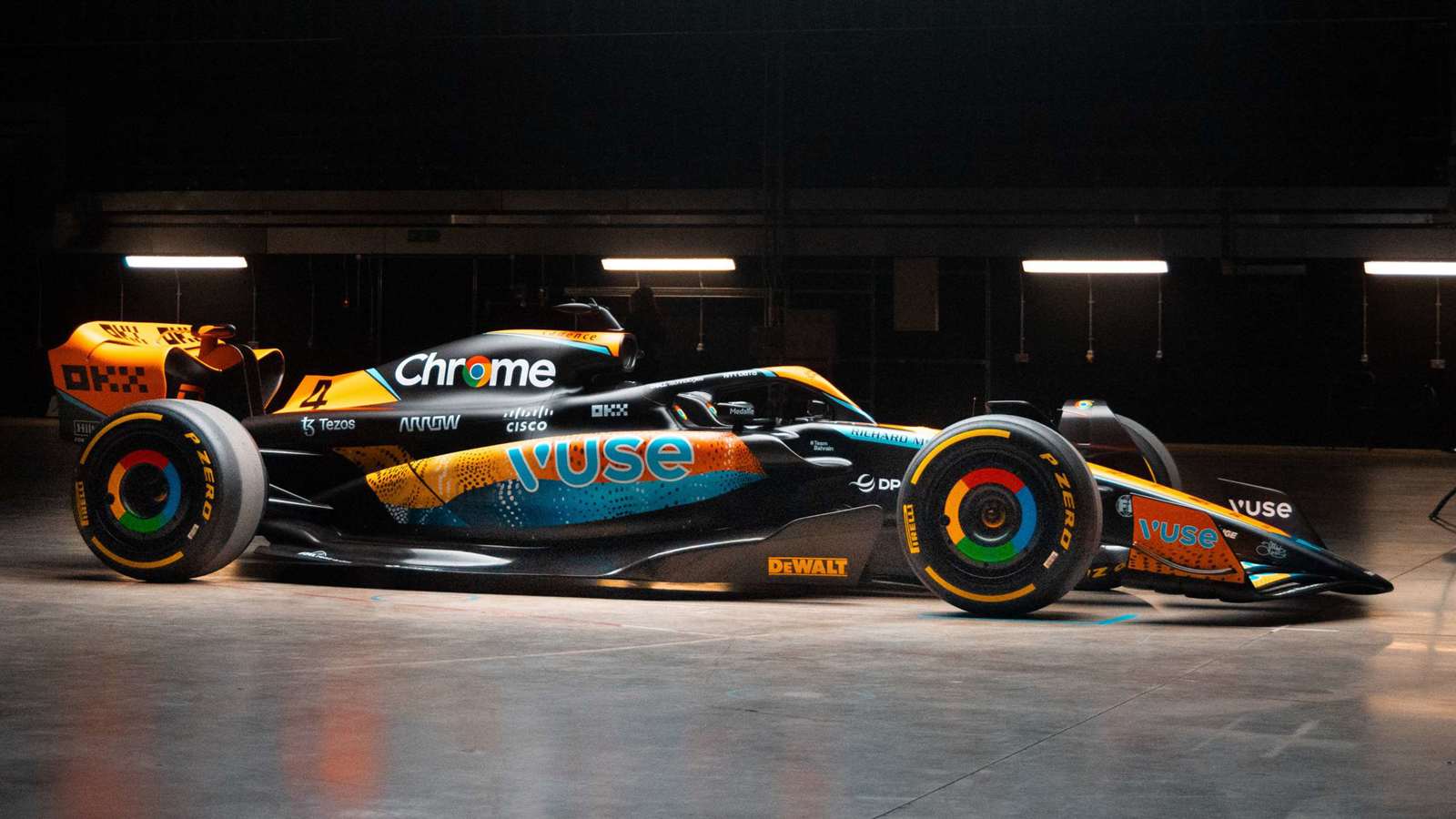The photograph features a sleek Formula race car with an open cockpit design, showcasing a narrow housing for the driver and essential components, constructed from a material that exudes a glossy, plastic-like sheen. The car's primary color is black, accented with striking yellow and blue details. Prominent sponsors are visible on the body of the car, including large "Chrome" lettering emblazoned in white, with the 'O' incorporating the multicolored Google logo. Other significant sponsors include Cisco, Aero, Tezos, and DeWalt, which appears towards the front in bold yellow. The VUSE logo, highlighted in blue with white outlines, is prominently displayed on the side and twice at the front with an orange background. The tires are notable for their P0 branding and colored interiors matching the Google Chrome palette. The car is situated on a shiny concrete floor in a dimly lit garage, illuminated primarily by horizontal fluorescent lights, which provide a stark contrast to the dark surroundings and highlight the car's vibrant details. The rear spoiler features the text "DKX" in black on a yellow backdrop, adding to the intricate visual appeal of the vehicle.